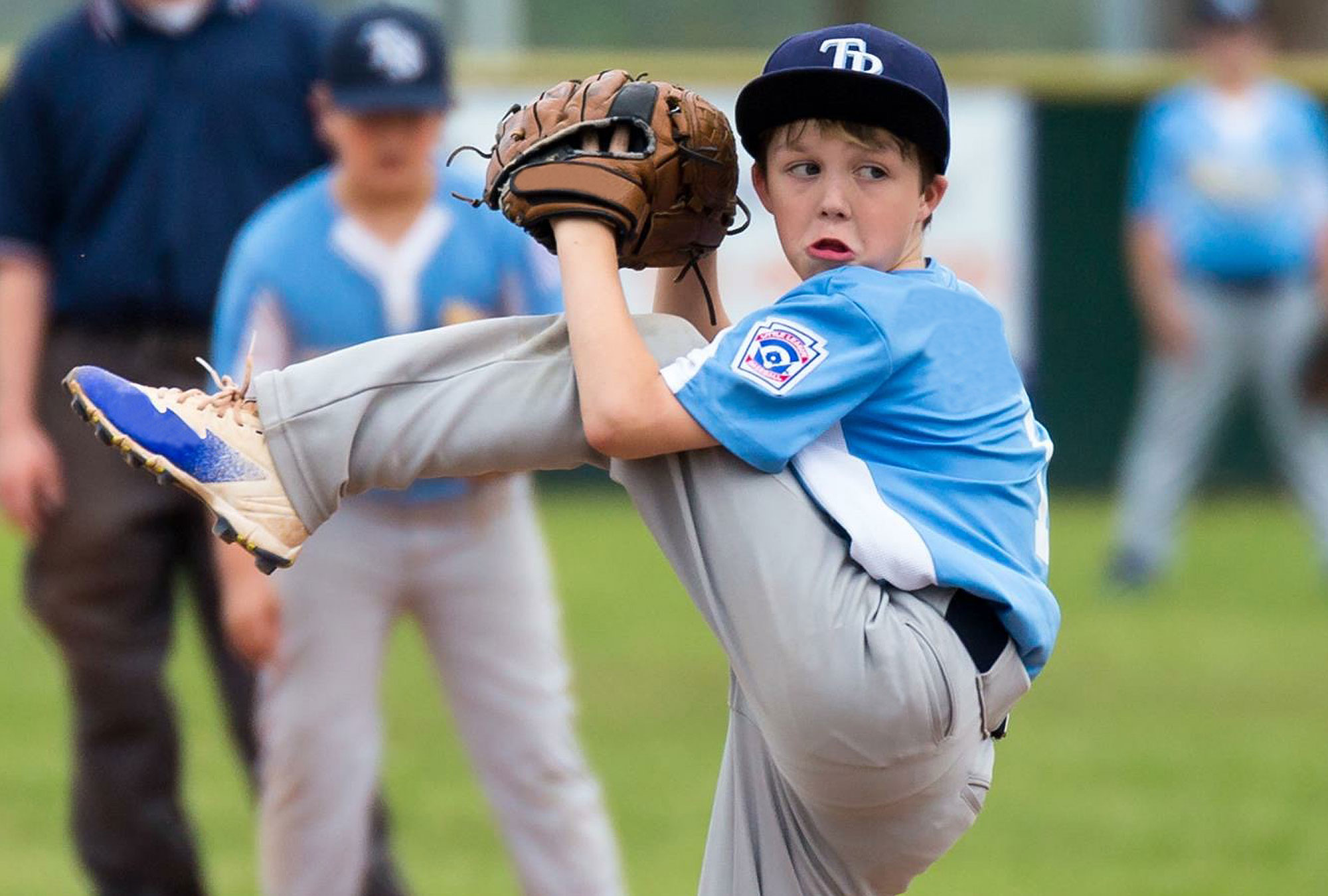The photo captures a moment during a kids' baseball game, focusing on a young pitcher in mid-throw. The boy is wearing a light blue jersey with white front, gray pants, and beige cleats with blue highlights on the toe. His jersey has a logo on the left arm, partially obscured, and he sports a blue baseball cap with white letters "TB" on the front. His pitching form is captured perfectly with his left leg raised high, left arm up with a large reddish-brown glove featuring a black stripe near the front, and his right hand tucked into the mitt. The boy's intense expression is turned to the right, fully concentrated on the game. In the blurred background, there are two other players dressed similarly, one to the right standing with legs apart and another to the left. Additionally, a man with a white beard, dark blue shirt, and brown pants, likely a coach or umpire, is also visible but out of focus. The setting is a grassy field with a green wall above the outfield fence, filling the scene with vibrant, natural colors. The attention is centered on the pitcher, embodying the spirit and determination of youth baseball.